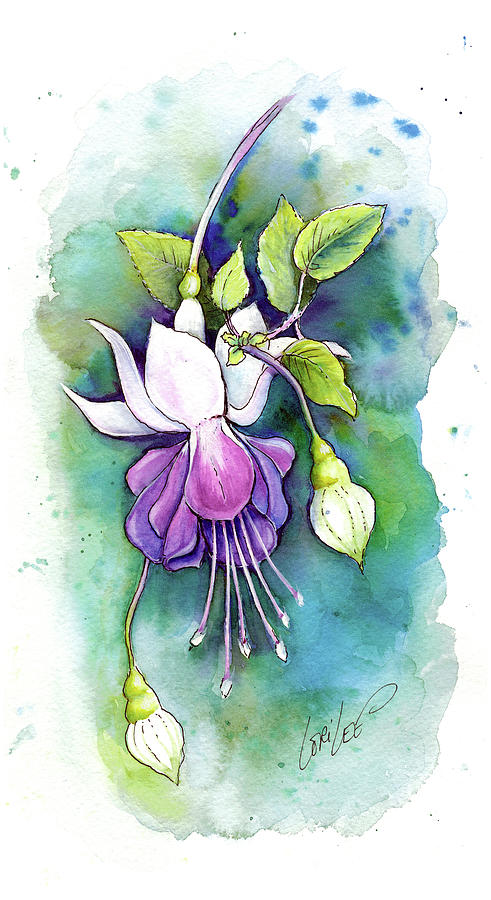This hand-drawn illustration by Lori Lee, rendered in watercolor, depicts a fantastical drooping flower. The flower showcases a gradient of purple hues, transitioning from dark purples near the bottom to lighter shades near the top. The stem, which curves from the top of the image, is a similarly colored mix of purples and whites, anchored by a green bulb. The flower's head features multiple antenna-like tentacles extending outwards, each ending in wider blue tips. Additionally, there are several bulbs nestled among the leaves around the flower, which appear to be heavy and hanging down. The background consists of a dreamy blend of blue, green, and white splotches, creating a cloud-like effect. The artist's signature can be found in the bottom right corner, enveloping the flower in an ethereal ambiance.